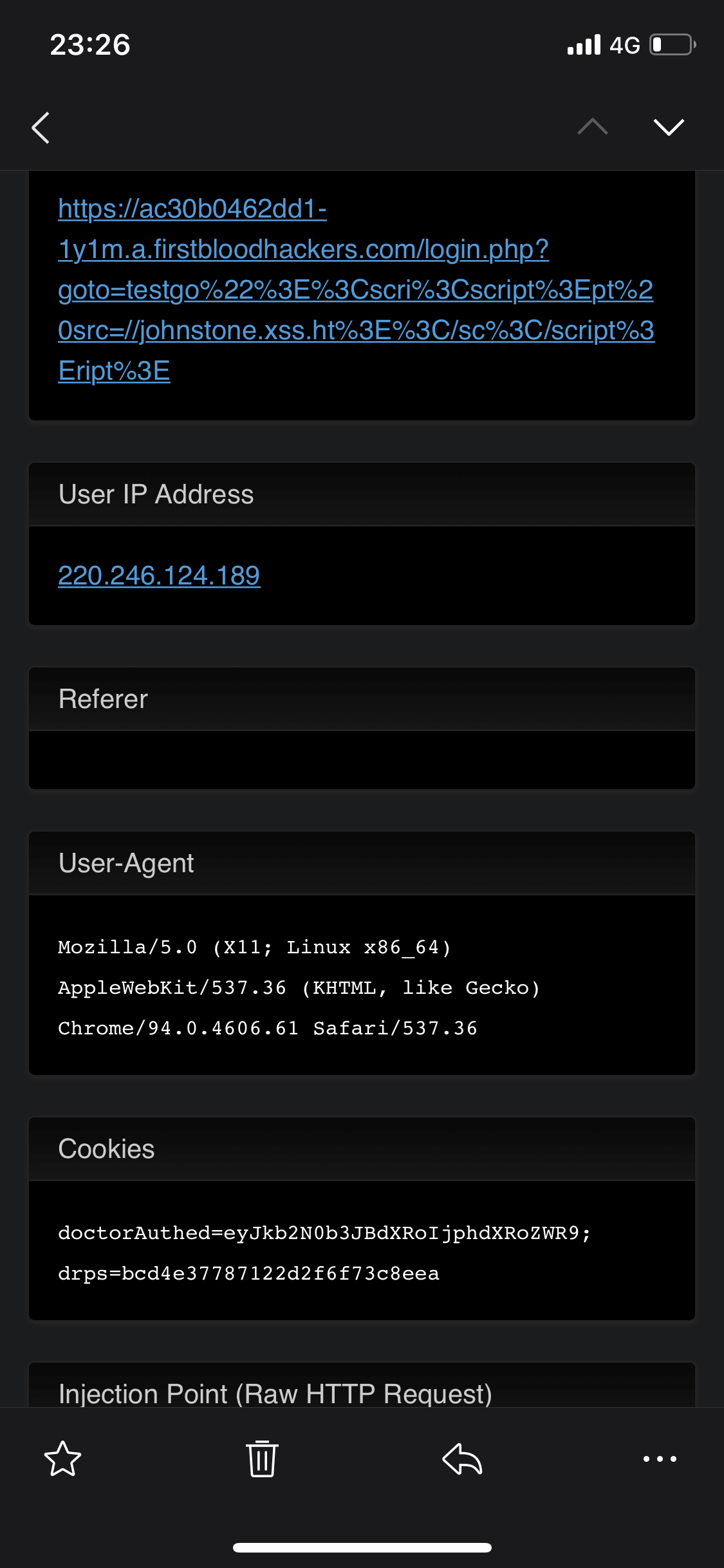The image appears to be a screenshot from a smartphone. The background is predominantly black. In the top left corner, the time displayed is 23:26. On the upper right corner, the status bar shows four signal bars, "4G" connectivity, and a battery level estimated at 25%.

At the top of the screen, there is a clickable blue hyperlink containing a complex string of characters, which begins with the URL "a.firstbloodhackers.com/login" followed by an assortment of additional letters, numbers, and symbols. Below this URL, the text "User IP Address" is displayed in white font. The IP address "220.246.124.189" is highlighted in blue directly beneath this.

The rest of the content on the screen is presented in white text. It starts with the label "Refer," followed by "User Agent," which is identified as "Mozilla/5.0" among other specifications including "AppleWebKit," "Chrome," and "Safari." Below this information, the word "Cookies" is listed alongside another website. Towards the end, the term "Injection Point" is followed by "raw HTTP request," suggesting this may be a technical screen related to web development or security monitoring.

Overall, the screenshot details various technical aspects such as network status, user IP address, user agent information, and web requests.